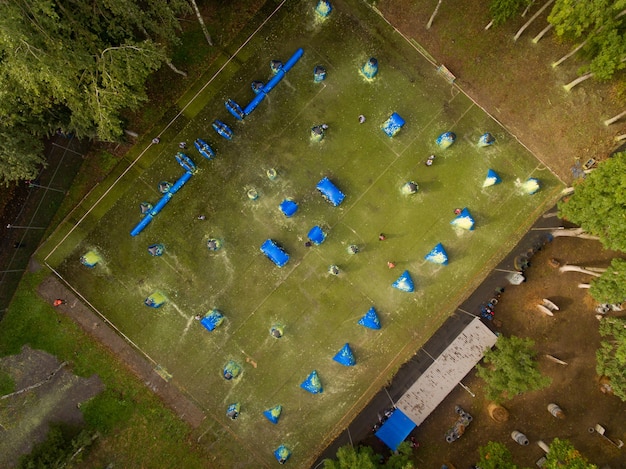This aerial image captures a paintball arena, seamlessly nestled within a dense forest. The field, resembling a tilted green rectangle about the size of a tennis court, is distinctly marked with various blue inflatable structures - squares and triangles - set out in specific locations. These blue items, which sport visible yellow paint splatters, serve as cover for players during games. Several individuals can be seen walking around the arena, although specific activities are hard to discern due to the height of the shot, suggesting it was taken by a drone or plane.

The left side of the arena is bordered by a fence, beyond which a dense cluster of trees is visible, showcasing both trunks and leaf canopies. Additionally, the bottom right corner of the field houses a cable spool on its side and open-topped barrels or containers, adding to the functional aspect of the location. A dugout-like viewing area is positioned to the right, illustrating a space for spectators. Outside the rectangle, a small white rectangle and a smaller blue square can also be observed. This image provides a well-rounded view of the arena, emphasizing its forested surroundings and detailing both the setup and some equipment present on-site.